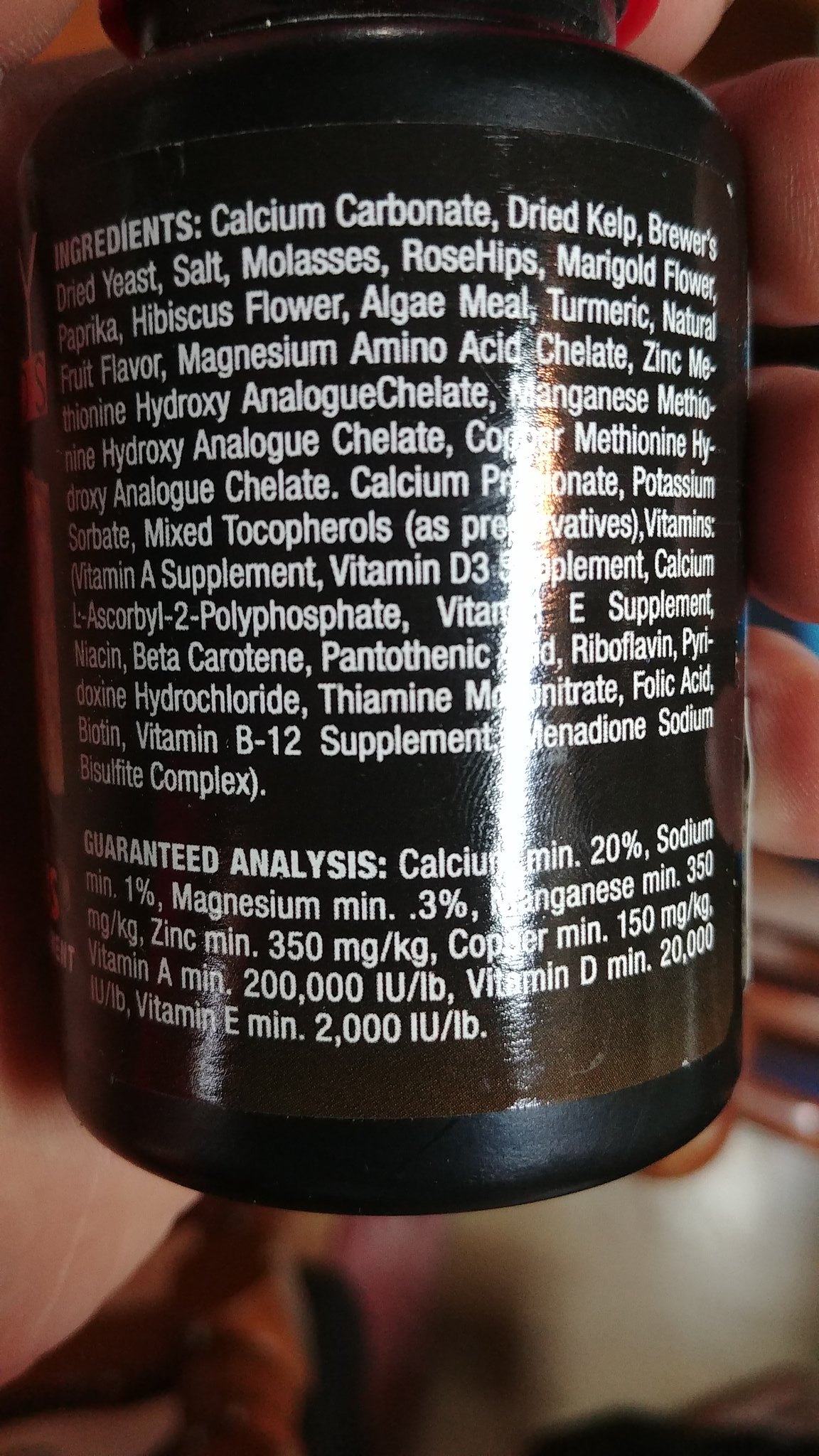The image features a dark-colored bottle, possibly black, containing a dietary supplement. The label on this opaque bottle is a combination of black and brown hues, with text written in white for contrast and readability. The back of the bottle is in focus, displaying a detailed list of ingredients. Some of the key components listed include calcium carbonate, dried kelp, yeast, salt, molasses, rose hips, marigold flower, paprika, hibiscus flower, algae meal, turmeric, natural fruit flavor, magnesium amino acids, zinc hydroxyanalog chelate, and manganese.